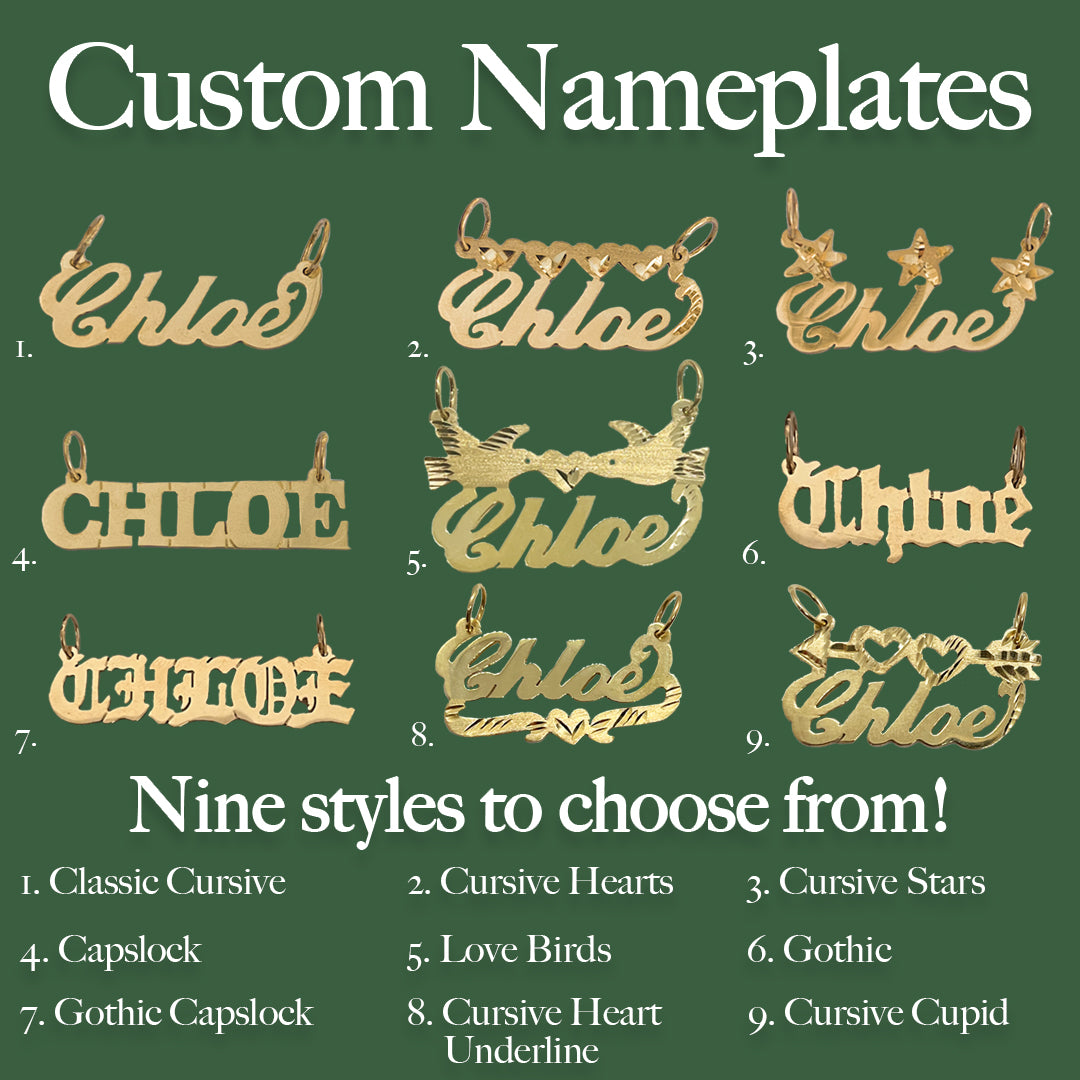The image is an advertisement displaying custom gold nameplates set against a green background with white text. At the top, it prominently says "Custom Nameplates" in big, white letters. Below this heading, nine different versions of the nameplate, all showcasing the name "Chloe," are displayed, each numbered 1 through 9. These nameplates are gold-colored and feature various fonts and embellishments. Among the styles, one of them, numbered 2, features a script font with a row of hearts above the name, whereas another, numbered 7, displays a gothic capital letter font. Additional embellishments include stars, hearts, lovebirds, and cupid icons. The styles named at the bottom of the image include classic cursive, cursive hearts, cursive stars, caps lock, lovebirds, gothic, gothic caps lock, cursive heart underline, and cursive cupid. The gold nameplates appear to be designed to be worn as jewelry or possibly used as decorative door signs, suggested by the inclusion of rings on either side of each nameplate.